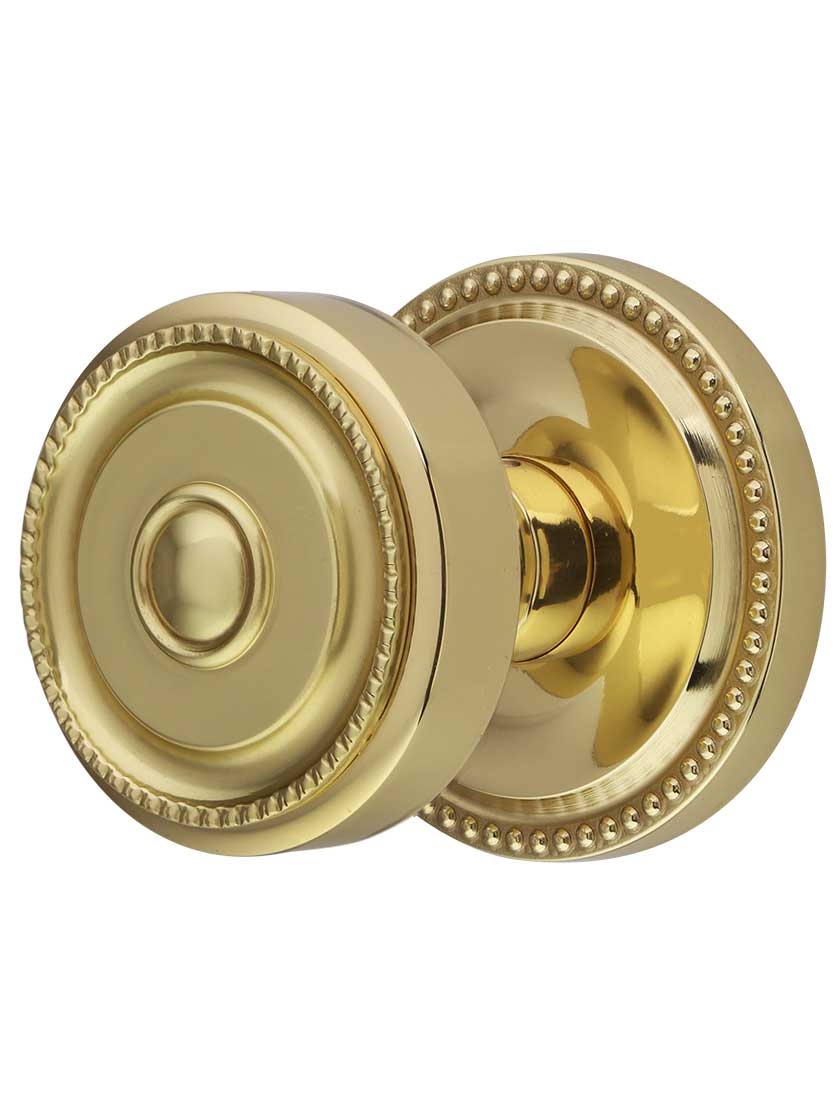The image features a detailed, golden doorknob set against a plain white background. The doorknob is perfectly round and intricately designed with a series of concentric patterns. The outermost design appears scalloped, resembling decorative indentations. Inside, there's a smooth round edge with an etched circle in the middle. The base, slightly larger than the handle, mirrors the concentric designs and is adorned with bead-like studs encircling it. A central tube connects the handle to the base, both elements finished in a lustrous golden hue. The glossy surface catches the light, enhancing its elaborate and ornate appearance.